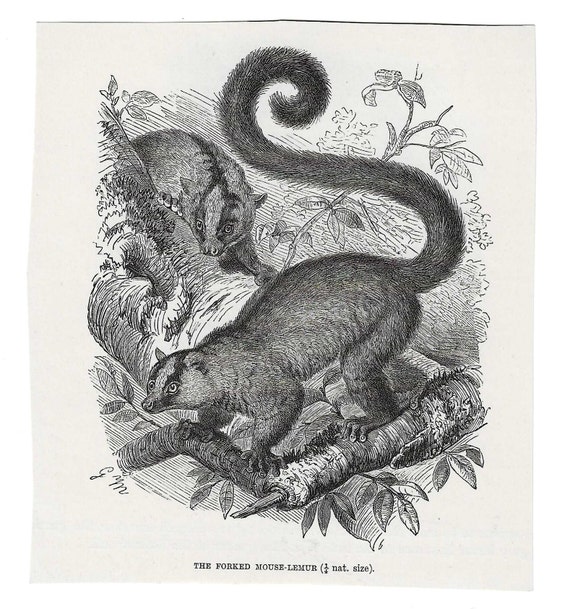This detailed black and white etching, a print of an old illustration, depicts two Forked Mouse Lemurs in their natural habitat. Labeled "Forked Mouse Lemur" at the bottom center, the scene shows one lemur with a long, spiraled tail navigating a tree branch, while another lemur peeks around the trunk, gazing directly at the viewer. Surrounding the lemurs are intricate depictions of leaves and branches. The artwork is signed with the initials "GM," emphasizing its classic styling and monochrome palette.